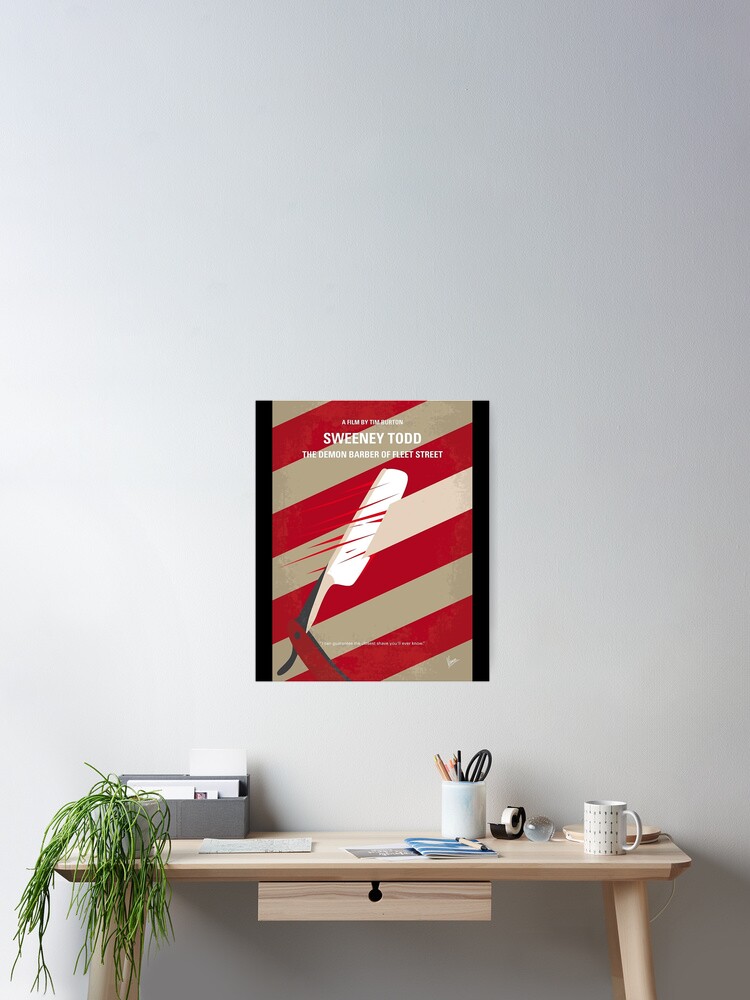This color photograph showcases a meticulously arranged light wood desk set against a white wall. The desk features a front drawer and is adorned with various items: a long-necked, adjustable white lamp; a cup filled with pencils and pens; a coffee mug; a tape dispenser; and an organizer box with papers sprawled across the surface. A striking visual element is a lush green plant overhanging from the left side of the desk, adding a touch of nature to the setting. Dominating the wall above the desk is a poster for the film "Sweeney Todd: The Demon Barber of Fleet Street" by Tim Burton. The poster has a bold red and tan striped background, with two black stripes flanking the sides and a straight razor at the center, depicted with a red handle and blood detail, creating a dramatic focal point.